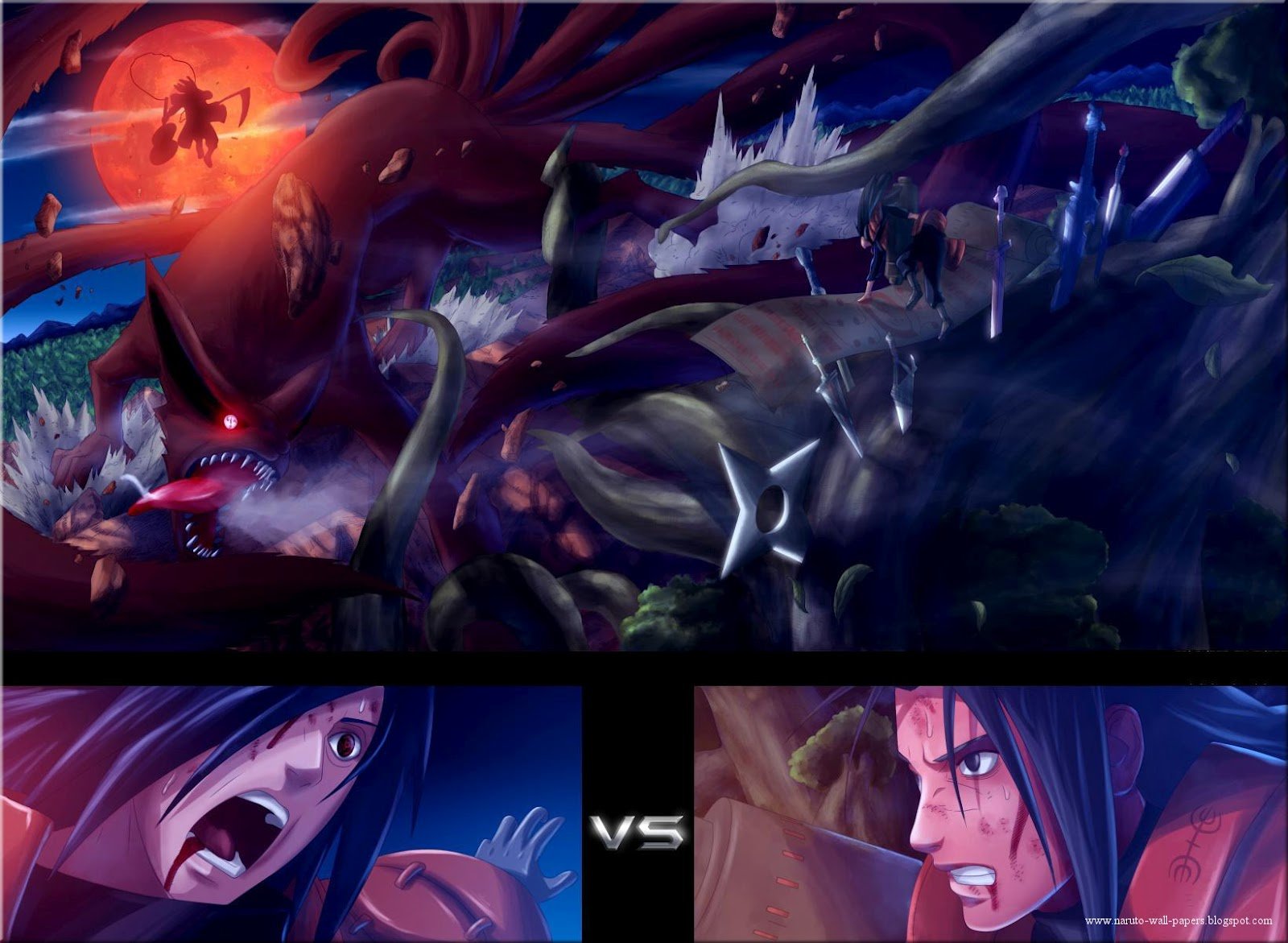The image, seemingly a scene from a video game, is split into three sections. The main, larger rectangular graphic at the top depicts an intense and ominous battle scene. Prominent in the background is a giant beast with sharp teeth and its tongue hanging out, accompanied by an eerie figure hovering in front of a large moon, casting a sinister vibe over the landscape. The sky around them is filled with reds and browns, adding to the menacing atmosphere. In the foreground, a four-legged creature stands on a broken landscape littered with swords and other weapons, suggesting a fierce battle. The creature is surrounded by cooler tones of blues, greens, and lighter browns, providing a stark contrast to the darker background. 

Below this main image are two smaller rectangular images placed side by side. To the left, one image shows the main character in distress, mouth agape, while the one on the right depicts the same character looking fierce, both battered and with blood dripping from their mouths. Between these two warriors, the text "VS" (versus) emphasizes their imminent confrontation. The characters wear brown armor, with their hair appearing black or blue, enhancing their rugged and battle-worn appearance. At the very bottom, there's a partly visible website URL, likely wallpaper.blogspot.com, hinting at the source of this dramatic and vividly detailed image.